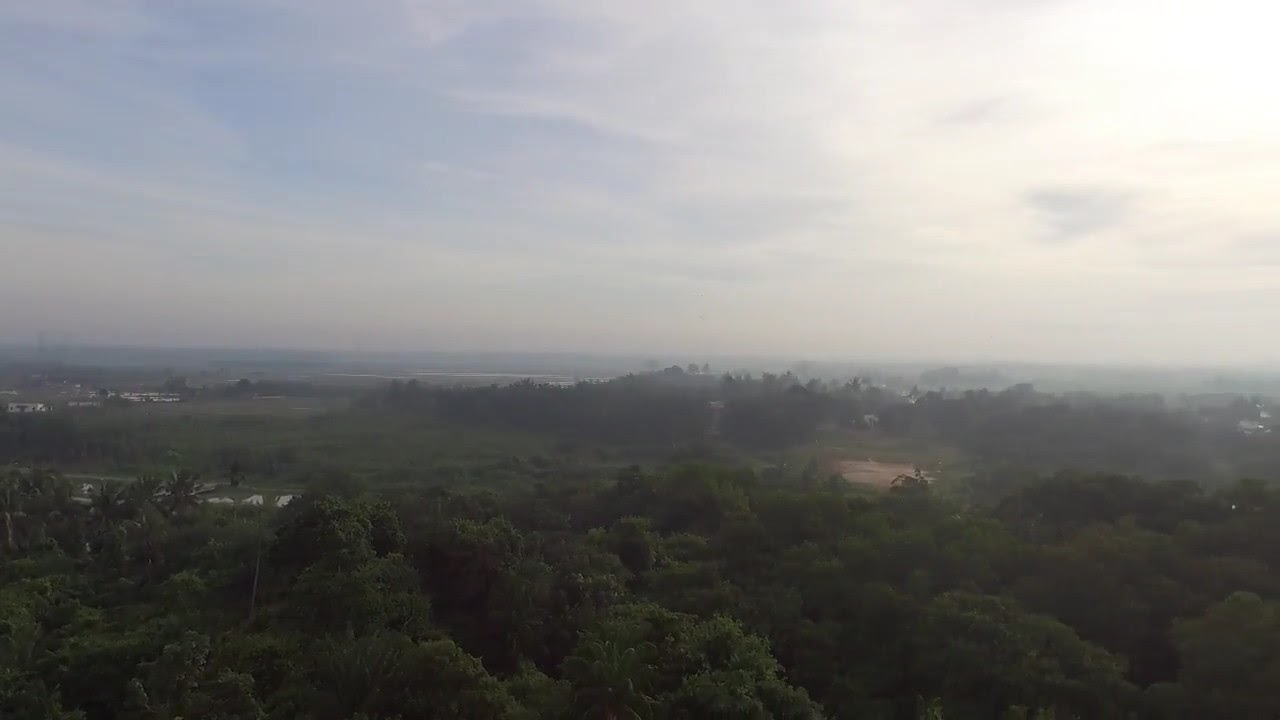The image depicts a vast expanse of trees stretching towards a hazy, smoky horizon, enveloping the middle part of the frame. The tops of the trees dominate the foreground with a mix of green foliage. Wispy, grayish clouds cover the mostly cloudy sky, with the sun's glow faintly visible through the clouds in the upper right corner, lending a subdued light to the scene. To the middle left of the image, a cluster of buildings—potentially houses, farmhouses, or industrial structures—barely break through the greenery. Their exact nature is indistinguishable due to the height from which the photo was taken, possibly from a drone or a tall building, as it offers a high vantage point, though not as elevated as an airplane. On the middle right, there's a noticeable brown patch, likely sand, dirt, or rocks, contrasting with the lush surroundings. In the distant background, there is ambiguity—what appears to be either water, mountains, or perhaps more forest, shrouded in mist or smoke, which blurs the line between land and sky, adding to the enigmatic atmosphere of the image.